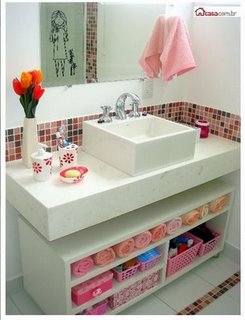The image depicts a modern bathroom characterized by a predominantly white color scheme with subtle accents of color. The walls are crisp white, matching the sleek, white countertop and vanity. The vanity features two sections separated by a small gap, with the upper section hosting a square, white sink that sits on the surface, enhanced with chrome fixtures. Below the sink area, there is a shelving unit.

The floor is adorned with white tiles interspersed with small, colored tiles forming a discreet pattern. These tiny colorful tiles continue as a decorative strip along the bottom of the wall, ending where it meets the countertop.

On the countertop, various items are arranged meticulously, including a rectangular mirror reflecting what appears to be a shower curtain illustrated with a playful drawing of a girl and a dog. The countertop also hosts a white vase filled with vibrant orange-red flowers and several white cups accented with red decorations. Other knick-knacks such as a soap dish and another cup add to the bathroom's organized charm. 

A soft pink towel hangs neatly, contrasting gently with the surrounding white elements. Beneath the countertop in the shelving unit, there are neatly rolled, pastel-colored towels and a collection of baskets, maintaining the bathroom’s tidy and welcoming appearance. The overall impression is of a carefully curated and clean space with thoughtful touches of color and decor.